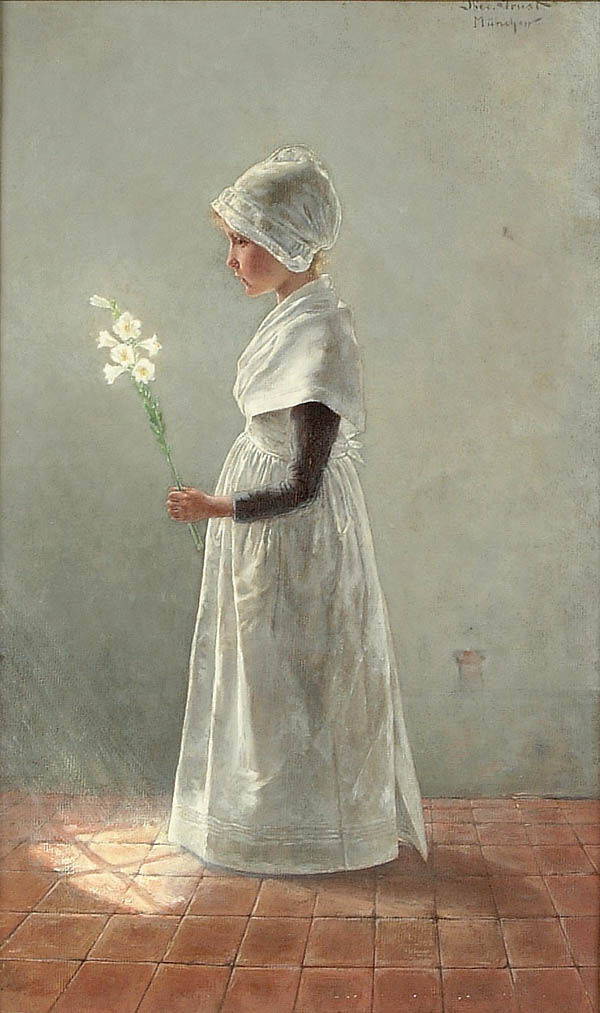The painting depicts a young girl standing against a gray wall, her figure illuminated by sunlight streaming onto a red brick floor at her feet. She wears a traditional bonnet, white and snugly covering her blonde, likely curly or frizzy, hair that peeks out underneath. Her attire consists of a white apron-like dress over a black, long-sleeved tunic, reminiscent of Pilgrim or Puritan clothing. Facing left, she holds a bouquet of white flowers, possibly lilies or daffodils, with green stems. The meticulous detail of the bricks shows orderly rows and columns, accentuating the neatness of the scene. In the top right corner, there is a small, somewhat illegible signature of the artist.